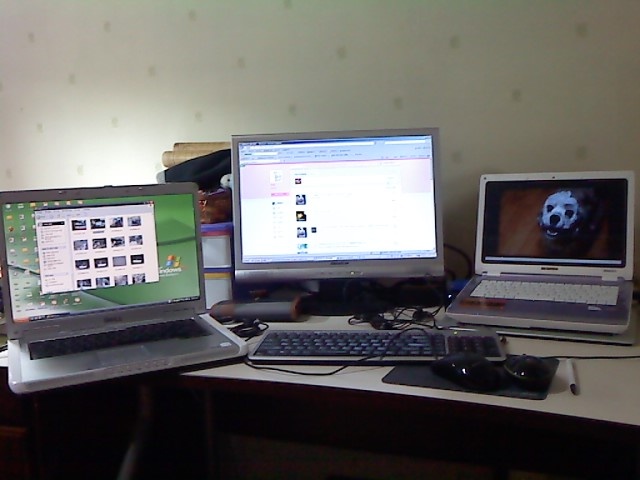The photograph displays a beige workdesk, matching the beige walls adorned with small light gray dots. On the desk, from left to right, are three electronic devices: two laptops and a monitor. The first laptop on the left is silver, with black inlay keys and a Windows XP background depicting green rolling hills, an orange start menu, a dark blue taskbar, and icons neatly arranged on the left side. It appears to have an open window showcasing numerous files, likely images.

At the center of the desk is a small, silver monitor connected to a silver keyboard with black keys and a black number pad. This setup is powered by a desktop computer. On the monitor's screen is a webpage primarily filled with images, presented with a gray border to optimize loading speed. Adjacent to the keyboard are two black mice on a shared black mouse pad, and a white pen with a black tip lies nearby. Behind the monitor, some books and other office supplies are visible, reinforcing the setup's work-oriented nature.

To the right is the second laptop, white with a close-up background image of a black and white dog with a white face, its mouth open, revealing its black eyes and nose. The desktop's taskbar is gray. This laptop too features a mix of white casing and a silver top.

Overall, the workspace is equipped with various computers and peripherals, reflecting a multi-device setup designed for efficient handling of multiple tasks.